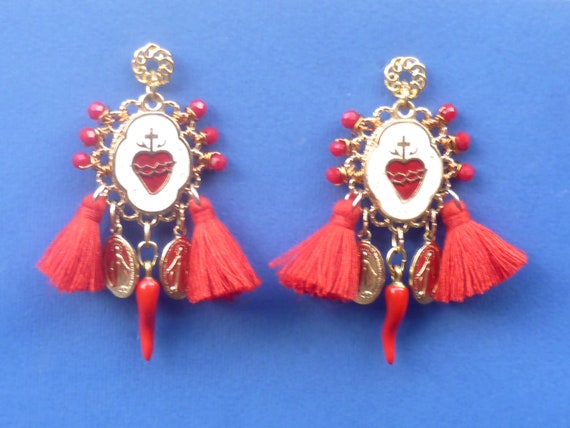This image showcases a close-up of two identical, ornate earrings set against a light blue background. Each earring features a decorative mixture of gold and white, with the central white oval frame containing a red element that resembles a strawberry or apple topped with a small cross. Below the central part, there are various intricate adornments including red chili pepper-like shapes, small coins, and little pom-poms. The earrings are embellished with gold appendages and red gemstones, and both earrings are detailed with red tassels. Despite the intricate design, the earrings clearly have clips at the top for attaching to ears, confirming their identity as earrings.